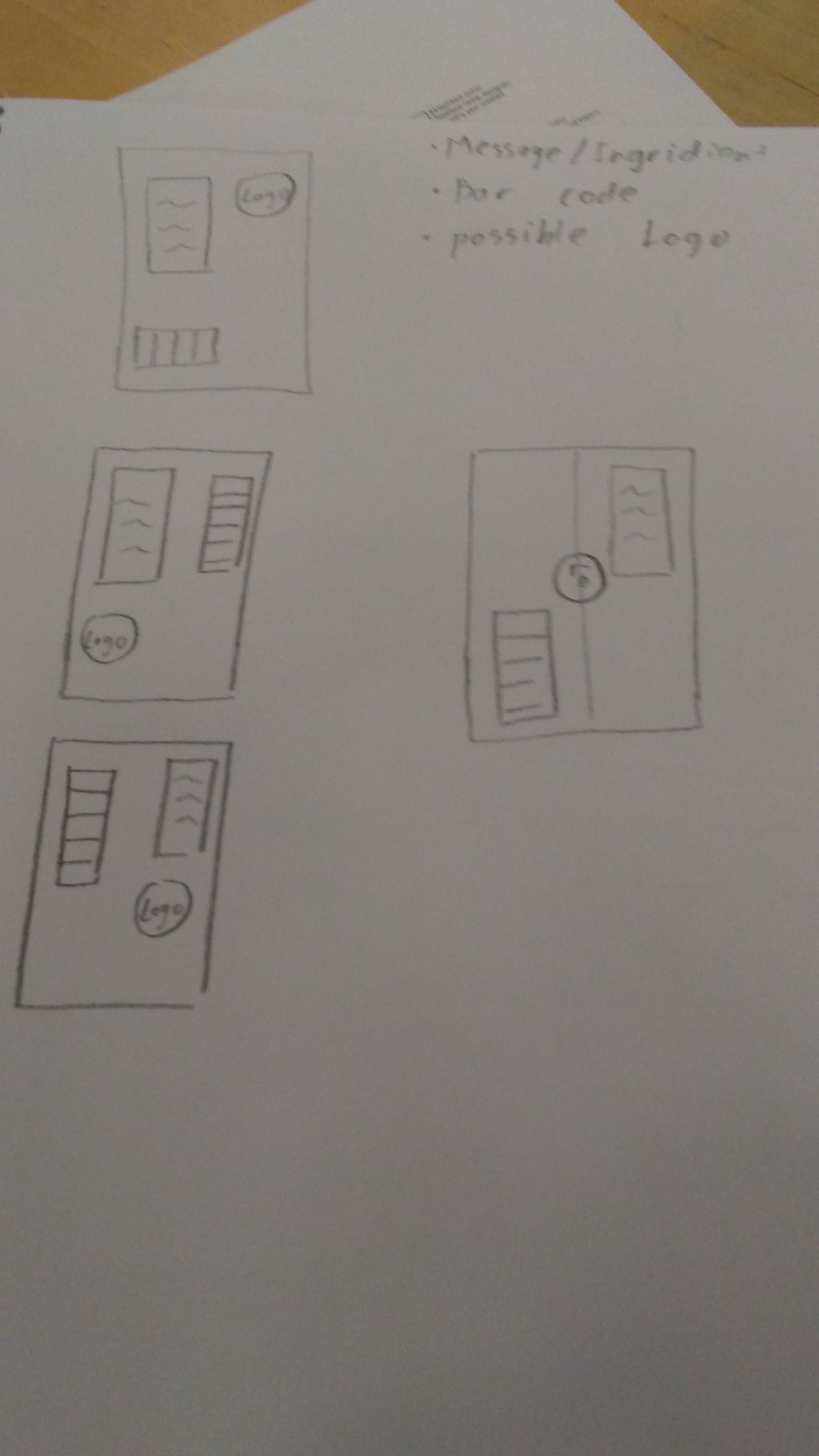In the image, a sheet of paper features a series of pencil-drawn sketches, presenting simplistic, preliminary designs possibly for vending machines. The layout includes four vertically oriented rectangles, divided into various sections depicting distinct elements of the proposed machines.

The first rectangle, situated at the top left, illustrates a design where a square, presumably displaying the items, is located at the top. Adjacent to this on the right side within the same rectangle, there is a circle labeled "logo". The bottom left section of this rectangle contains another smaller rectangle filled with vertical lines, indicating shelves or product slots.

The second rectangle on the upper middle left features another box with squiggles, likely representing items, to the left side. To its right is another box with lines, which might suggest a display or selection menu. The bottom left corner houses the logo while a box with horizontal lines appears nearby, denoting a different type of product presentation or slot.

In the third rectangle, positioned in the middle left, the logo appears on the right side of the bottom section this time. A box of horizontal lines is shifted to the left, and squiggles (items) move to the right, suggesting different organizational layouts of the vending machine's features.

The final rectangular sketch in the center right exhibits the logo positioned centrally with a line running through it, giving it prominence. Items are placed in the bottom left corner, while possible text is scribbled on the upper right, potentially denoting a brand's slogan or product description.

In the fourth and final rectangle at the upper right, a detailed layout includes bullet points reading "message/ingredient," "barcode," and "possible logo," indicating areas for displaying additional information about the products or the machine itself.